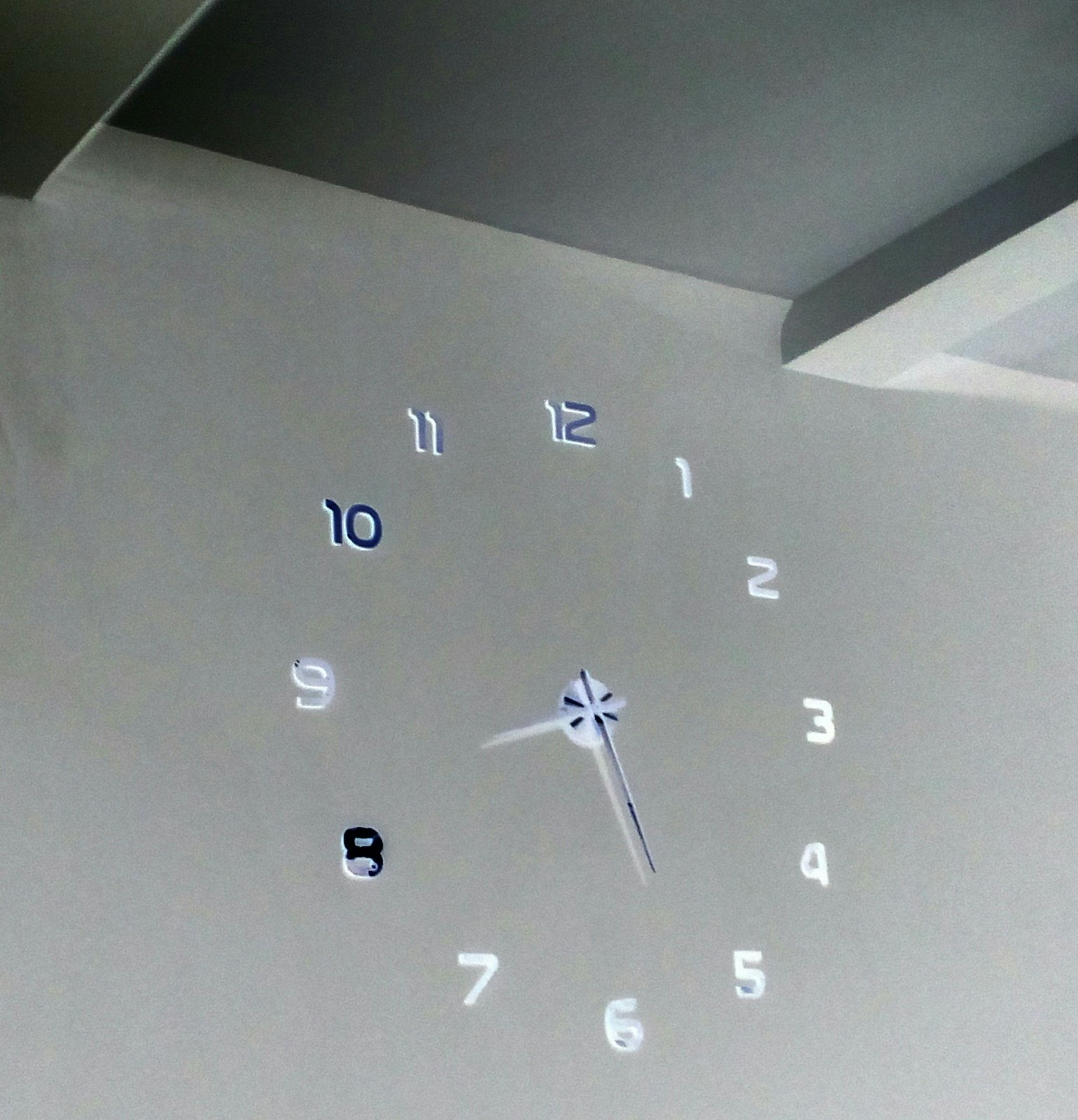The image features a frameless, borderless clock digitally projected onto a white wall, which appears grayish due to the play of shadows. The clock consists of bright white numbers 1 through 7, while the numbers 8, 10, 11, and 12 have a blackish-blue reflective quality. The numbers 11 and 12 show signs of wear, appearing gray and partially black, respectively. The clock hands, which are primarily white with black markings, indicate the time as approximately 8:27, with the smaller hand pointing between 8 and 9 and the larger hand between 5 and 6. The wall is topped by a gray ceiling with two visible white beams.